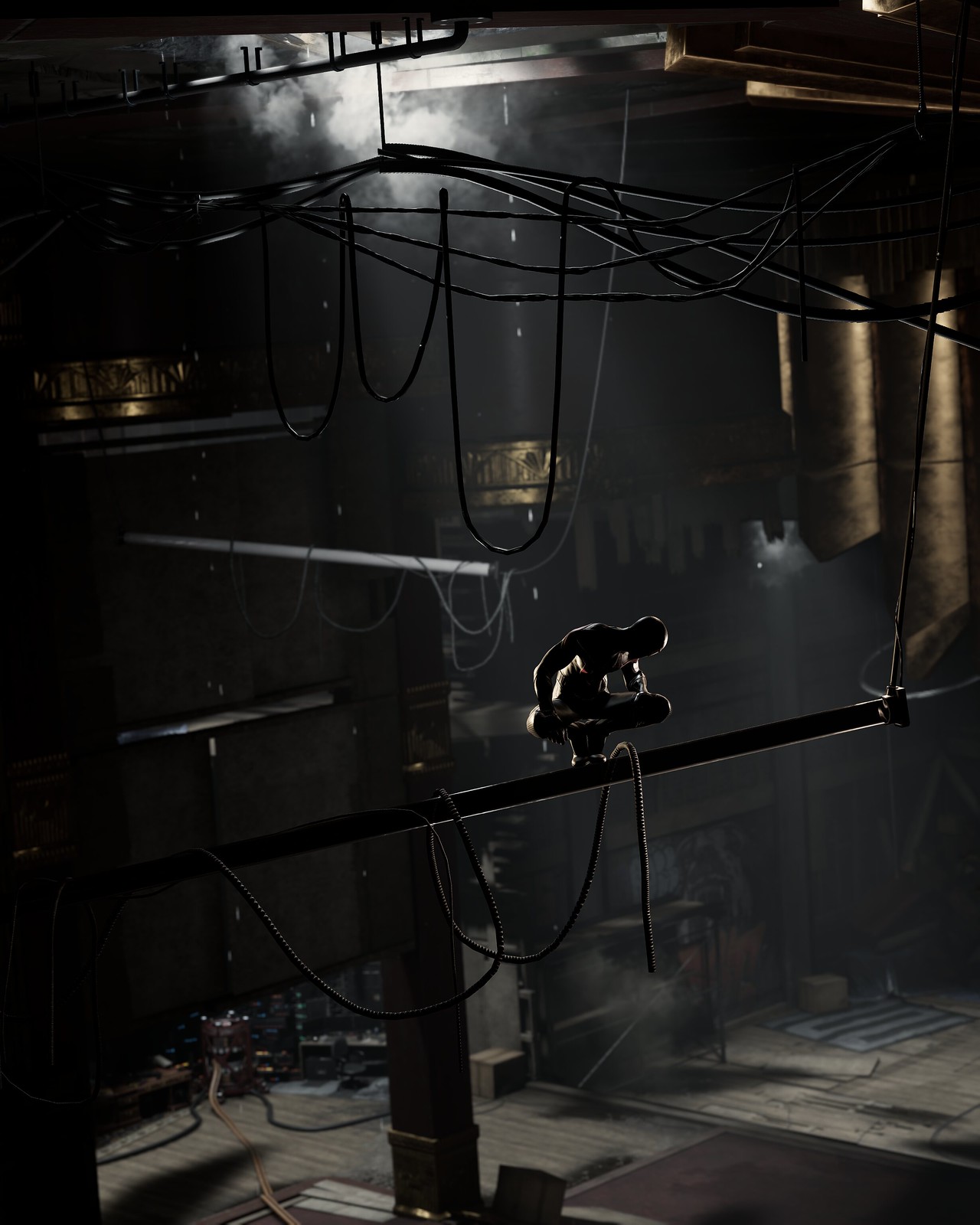In this very dark and atmospheric image, a Batman-like figure in a superhero outfit is crouched on a thick metal beam suspended across a large, industrial-looking room with a high ceiling. The room has a disused ambiance, emphasized by the various black and steel pipes of different sizes hanging down from above and looping around several times. Smoke lingers near a light source, adding to the gloomy atmosphere. Positioned prominently is a statue of a man bending down and looking over, atop a stand, surrounded by more metal and ropes hanging from the pipes. The floor is covered in gray square tiles, and there's a copper round bowl on a shelf beside what appears to be a fireplace. Additionally, a folded-up table lays inconspicuously on the tiled floor, contributing to the scene's overall mysterious and underground feel.